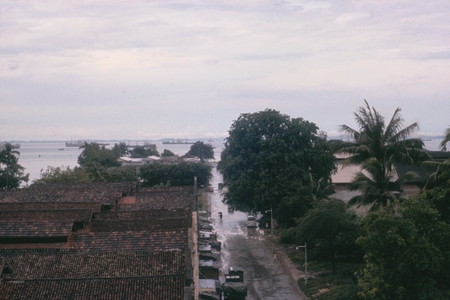An aerial photo captures a gloomy, overcast sky, indicative of recent or impending rain. Below, the image presents a tropical neighborhood with brick-colored rooftops, primarily on the left, and a road running through the center. The area is clearly experiencing flooding, as water seeps into the streets from the ocean visible in the distance, encroaching on houses and vehicles. On the right, dense clusters of green foliage and tall palm trees obscure parts of the view. Along the shoreline, several boats, including large fishing trawlers and smaller vessels, are moored, emphasizing the seaside location. The scene suggests a village grappling with the aftermath of a heavy storm.